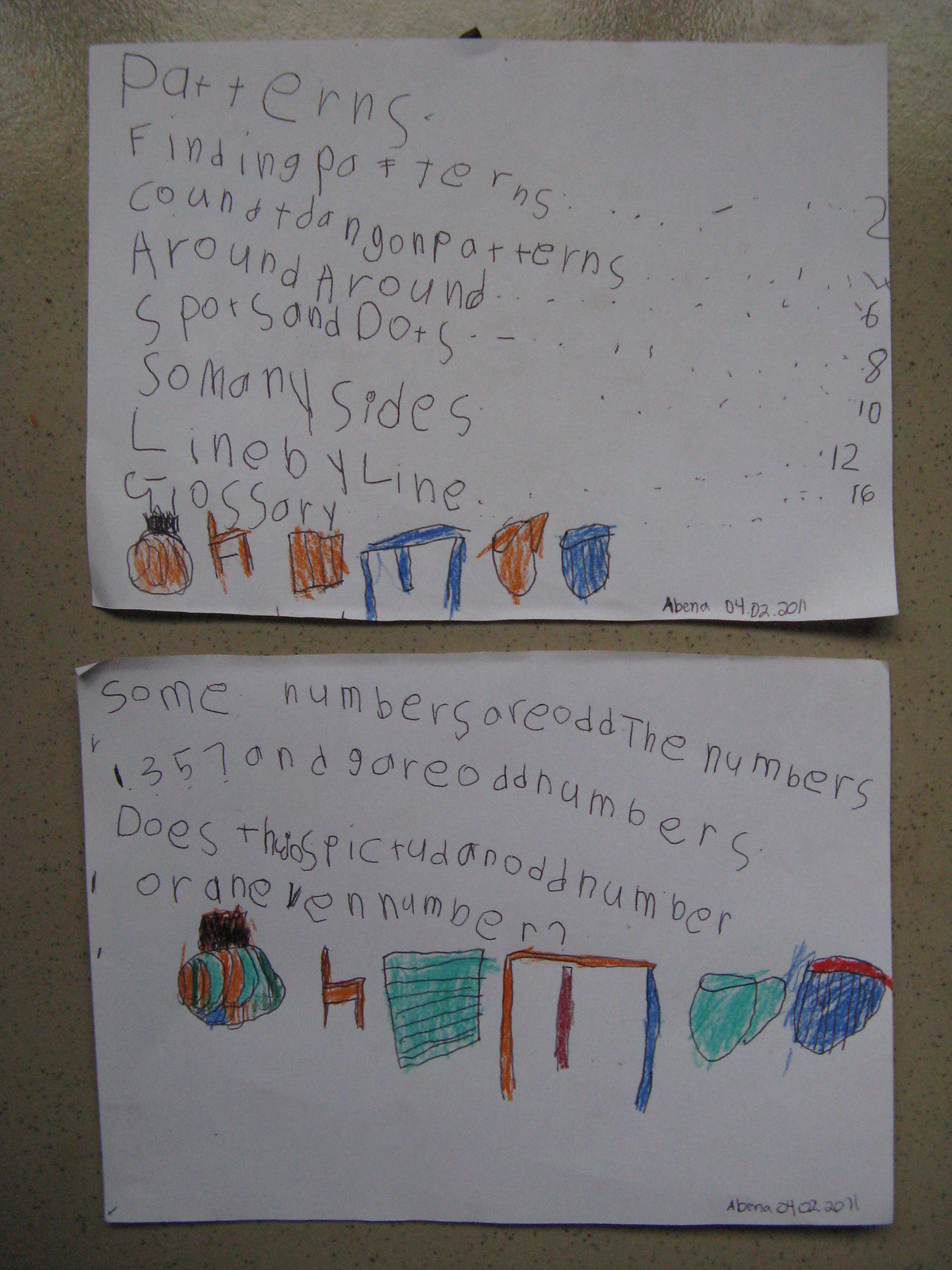This image shows two pieces of paper hanging on a browny-grey wall, both seemingly drawn and hand-written by a child. The top paper features a list with the words: "patterns, finding patterns, counting patterns, around around, spots and dots, so many sides, line by line, glossary," all scrawled in uneven, childlike handwriting. Below this text are illustrations that are hard to interpret but appear to include items such as a basketball, a chair, cups or mugs, and a table, arranged in a pattern. The bottom paper lists numbers, noting that 1, 3, 5, 7, and 9 are odd. It poses questions like "Does this pig have an odd number?" and "Orange van number," alongside more childlike drawings, which may depict a table, chairs, and a ball. The handwriting is challenging to decipher, with letters varying in size and alignment, typical of someone just learning to write. Both pieces are dated April 2nd, 2011.